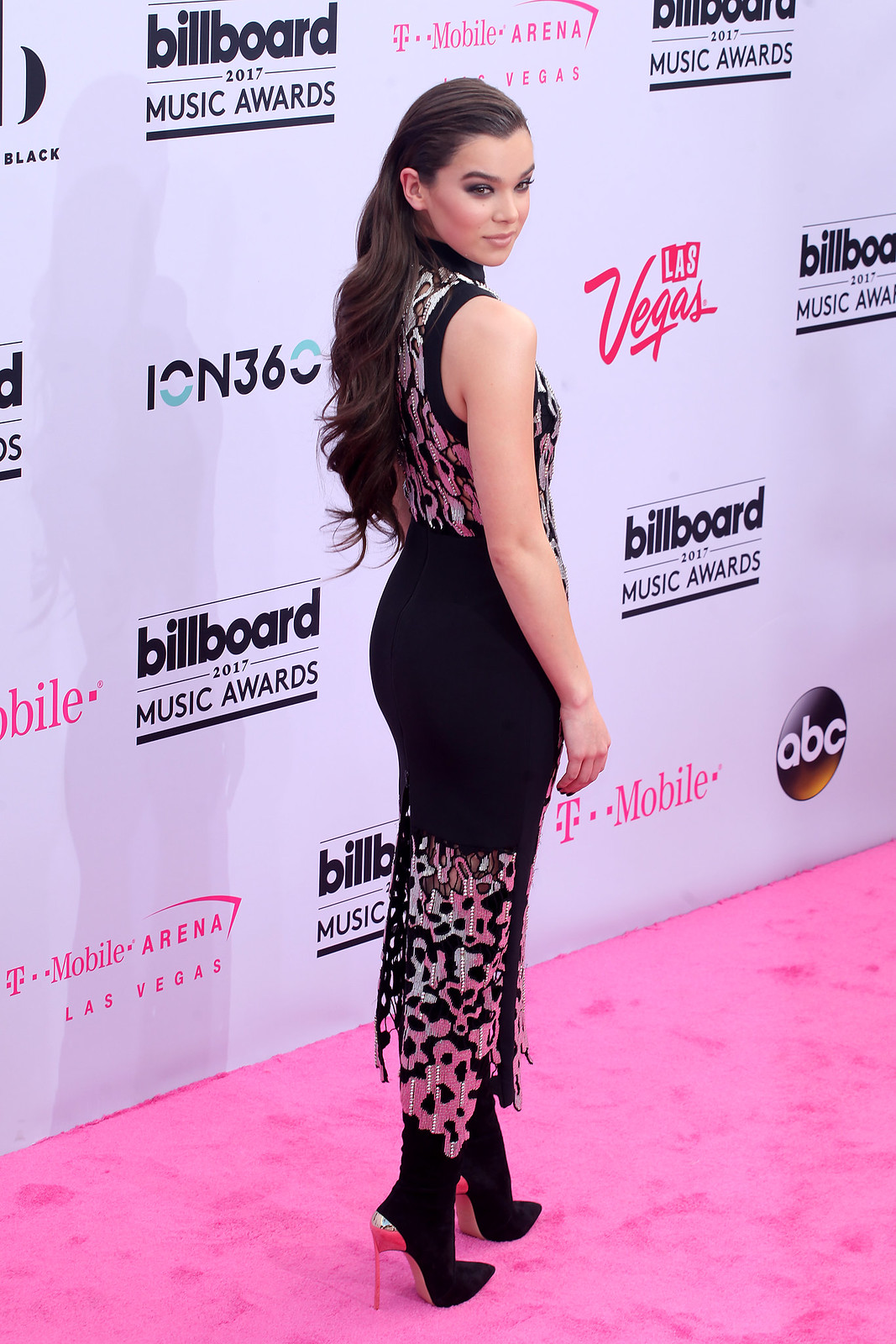A young woman with long, wavy, brown hair cascading down her back stands in front of a white billboard advertising the Billboard 2017 Music Awards, Las Vegas, ION36, and ABC. She wears a sleeveless, long black dress adorned with silver patterns and beads, which contrasts beautifully with her high-heeled black boots. The billboard behind her also features logos for T-Mobile and Mobile Arena alongside the text "Billboard 2017 Music Awards." The woman poses on a green carpet over a pink floor, turning slightly to reveal her right shoulder, her light skin illuminated by the scene. She confidently looks back towards the camera, capturing the essence of the glamorous event.